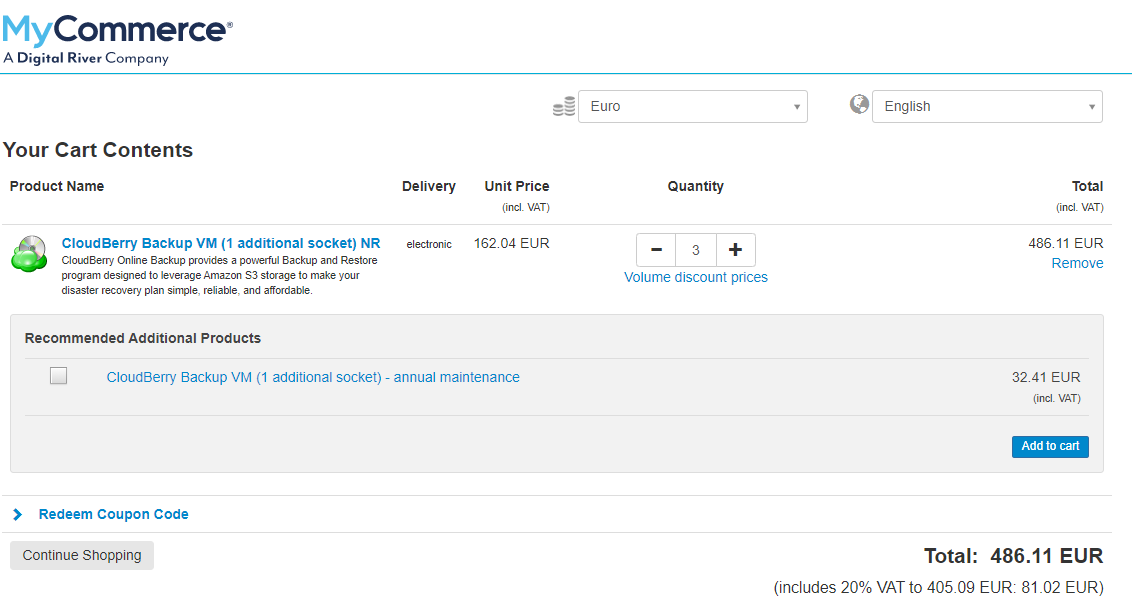The image depicts a detailed view of a MyCommerce shopping cart interface, which is associated with Digital River, a global e-commerce solutions company. The interface features a harmonious color scheme, with 'MyCommerce' highlighted in a light blue hue and 'Digital River Company' in a darker blue. 'Digital River Company' is prominently bolded, and beneath it runs a thin blue line extending horizontally across the interface.

Centered on the interface is a dropdown box for currency exchange rate adjustments and language selection, currently set to English. Moving towards the left, larger text reads "Your Cart Contents," followed by smaller text labeling each column, starting with "Product Name."

The featured product is "CloudBerry Backup VM," with its description in smaller black text and specific elements highlighted in blue. The description outlines that CloudBerry Online Backup offers a robust backup and restore program, which leverages Amazon S3 storage to make disaster recovery plans simple, reliable, and affordable.

Adjacent to the product description, there's a delivery option labeled "Electronic" and a unit price listed as €162.04. The quantity is set to three, with options to adjust using the plus and minus signs. Below this, in blue text, it states "Volume Discount Prices." The total price, including VAT, is €486.11, with the option to exclude VAT if necessary.

Recommendations for additional products, such as annual maintenance for €32.41, are presented below, with an "Add to Cart" button beside them. There's also a space to redeem a coupon code and a "Continue Shopping" button. Finally, the grand total, inclusive of a 20% VAT, is prominently displayed as €486.11.